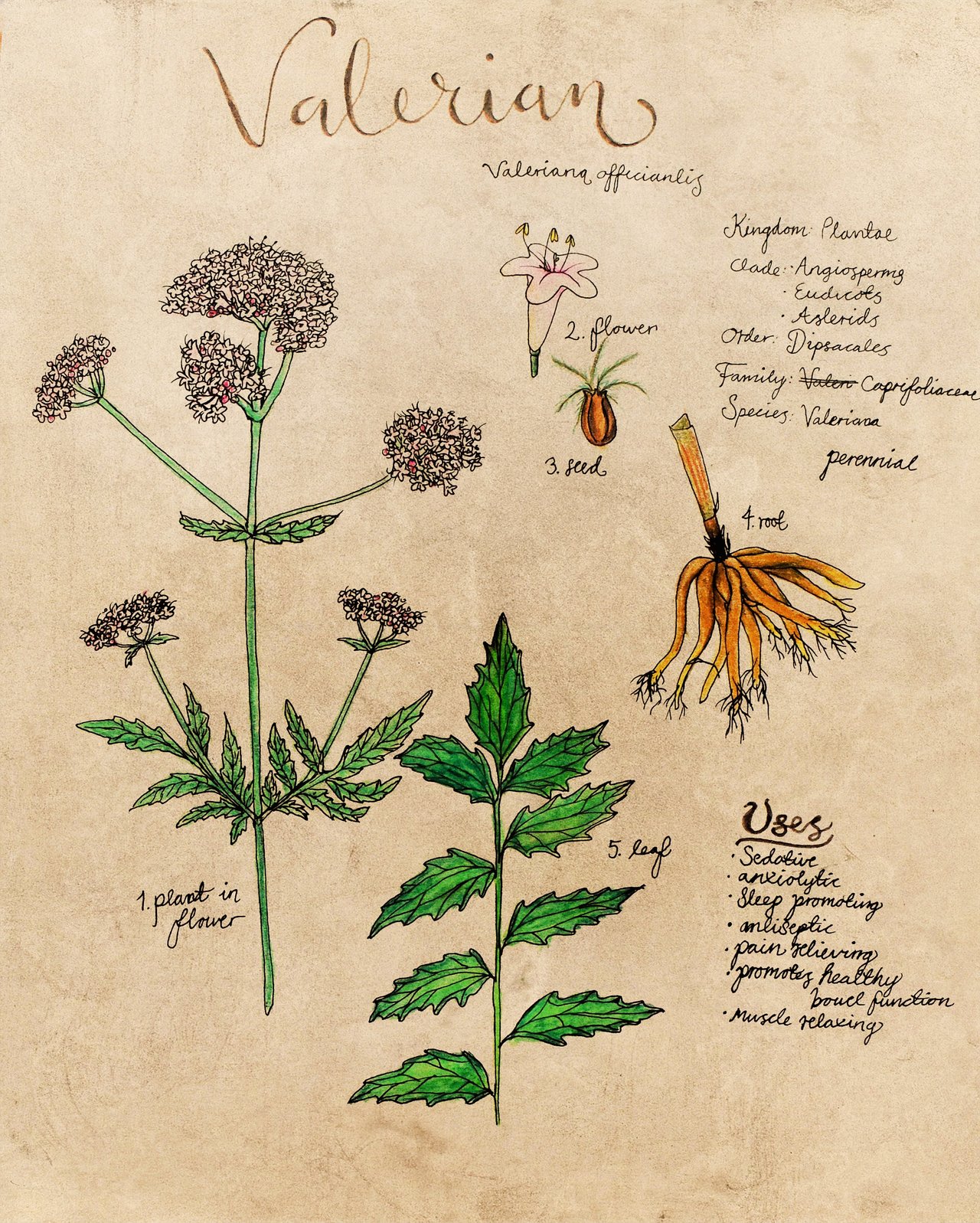This detailed, hand-drawn illustration of the medicinal herb Valerian (Valeriana officinalis) looks like a classic botanical illustration from horticultural books, featuring intricate drawings and informative notes. The drawing showcases the plant in several stages and parts: the main plant with its stem, branching leaves, and clusters of small white to purplish flowers; a close-up of the flower; a long stem with nine leaves; the root system depicted with orange hues; and a sprouting seed. The title "Valerian" is written in elegant cursive at the top, with the scientific name "Valeriana officinalis" beneath it.

Detailed botanical classifications including kingdom (Plantae), clade (Angiosperms, Eudicots, Asterids), order (Dipsacales), family (Caprifoliaceae, with a correction from Valerianaceae), and species (Valeriana), are noted in small cursive text on the right-hand side. The plant's perennial nature is also mentioned.

Under the "Uses" section, underlined and written in cursive, are the various medicinal properties of Valerian: sedative, anxiolytic, sleep-promoting, antiseptic, pain-relieving, promoting healthy bowel function, and muscle-relaxing. The entire illustration is delicately colored with pencil in green, brown, and pink, indicating a student's meticulous effort, further evidenced by some crossed-out words. This drawing captures both the plant's botanical complexity and its therapeutic significance.